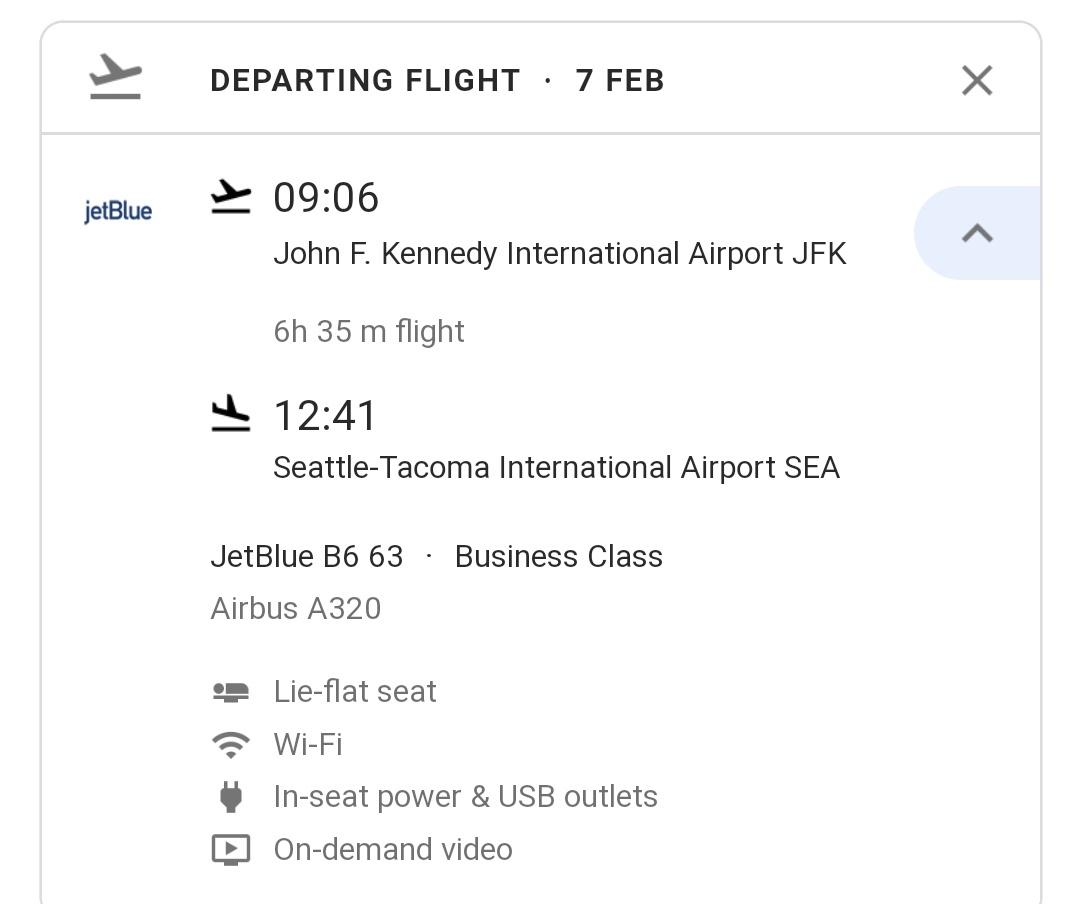### Detailed Flight Itinerary Caption

The image displays a detailed itinerary for an upcoming flight. At the top, there's a small icon of a grey plane taking off, with the text "Departing Flight 7 THEB" next to it. In the top right corner, there's a grey 'X' symbol. Below this, a grey horizontal line separates the initial section from the main details.

In the main section, the top left shows the airline "JetBlue" written in blue text. Next to it, there's a black icon of a plane taking off. Below this, the flight details are clearly specified: the departure time is "0906" from "John F. Kennedy International Airport (JFK)," with an estimated flight duration of "6 hours 35 minutes."

To the right of these details, there's a bluish upward-pointing arrow icon. Continuing down, there's another black icon, this one depicting a plane landing. Below it, the arrival time "1241" is shown at "Seattle-Tacoma International Airport (SEA)."

Further details include the flight information: "JetBlue B6-63 Business Class," on an "Airbus A320." At the bottom, there are four icons representing amenities provided during the flight:

1. **Lie-Flat Seat**
2. **WiFi**
3. **In-Seat Power and USB Outlets**
4. **On-Demand Video**

These features ensure a comfortable and connected travel experience.